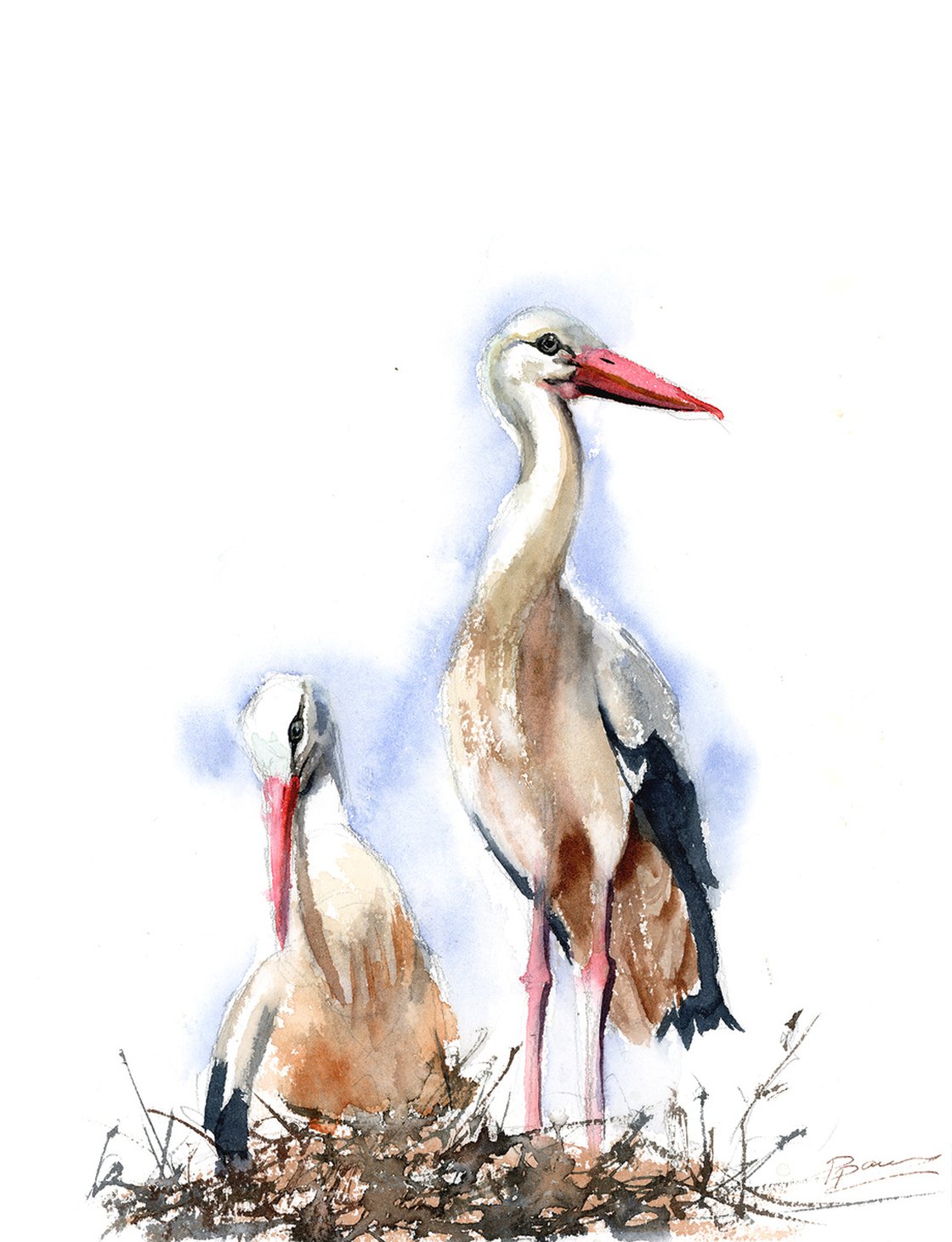This is an illustration of two large water birds, likely storks, rendered in a minimalist style. One of the storks is sitting down amidst rustling leaves and foliage, possibly nesting, while the other stands tall and alert beside it, appearing to be its mate. Both birds feature long legs, long necks, and distinct beaks with a peach-red hue. Their plumage showcases shades ranging from white to light brown. The background includes a subtle indication of sky, with a faint blue halo around the birds, suggesting an outdoor setting. The detailed foliage beneath them includes whites, grays, and browns, enriching the scene with natural tones. In the bottom right corner, there's a barely legible signature, possibly starting with a "B" or "P," though the exact name of the artist remains unclear.